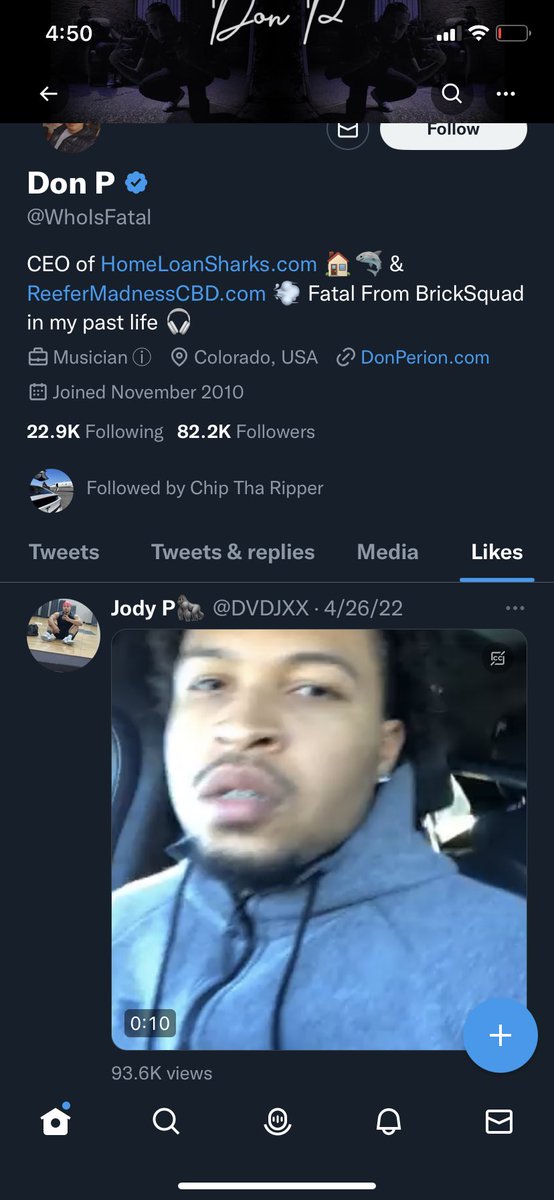This image appears to be a screenshot of a vertically oriented profile page on Twitter, now known as X, viewed on a smartphone. The profile belongs to a user named "Don P," featuring a somewhat unclear and dark cover image with handwriting across the top that reads "Don P." The profile name, "Don P," is accompanied by a verified blue checkmark, and the username is "@whoisfatal."

The bio section provides detailed information: Don P is described as the CEO of HomeLoanSharks.com, denoted with a house emoji, and ReeferMadnessCBD.com, symbolized by a smoke emoji. The bio also includes "Fatal from BrickSquad in my past life," alongside a headphones emoji, indicating a musical background. Don P is categorized as a musician based in Colorado, USA, with an external link to "Donperion.com." He joined the platform in November 2010.

At the time of the screenshot, Don P follows 22.9 thousand accounts and is followed by 82.2 thousand users. Notably, he is followed by Chip the Ripper, as indicated by a highlighted "followed by" section featuring Chip the Ripper's avatar.

The interface shows tabs for Tweets, Tweets & Replies, Media, and Likes, with the "Likes" tab currently highlighted. The first item in the Likes tab is a blurry 10-second video of a young Black man with a slight beard and mustache, wearing a blue zip-up hoodie or jacket. This video was posted by a user named Jody P.